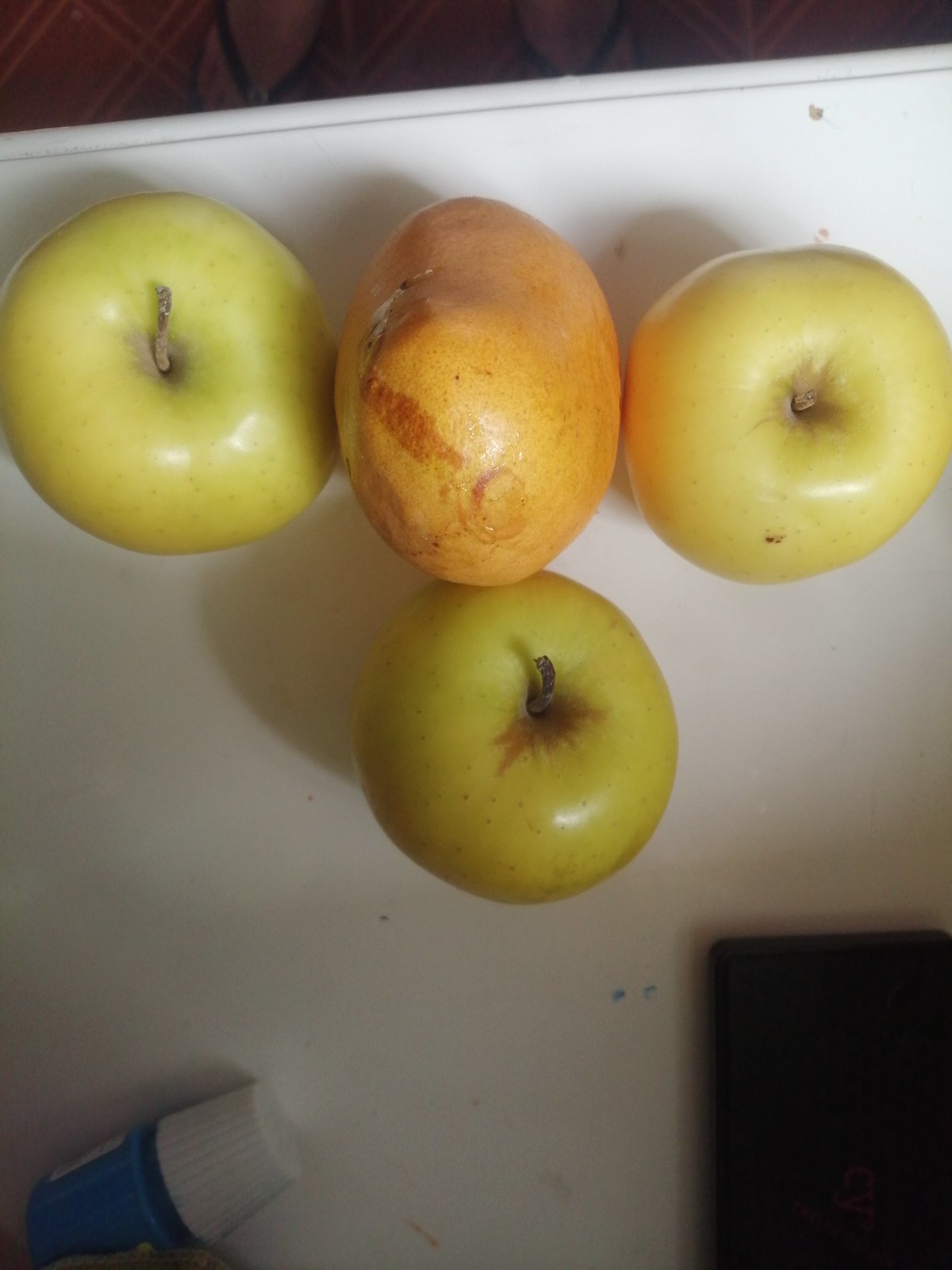In the top-down image, we see a collection of fruits arranged on a pristine white table. Prominently featured are three light green apples, each with a hint of brown around their stems. The apples form a triangular shape: one on the left, one on the right, and one at the bottom. At the center of this arrangement is a slightly deteriorated fruit, varying described as an old orange, pear, or mango, which has a reddish line on its surface, resembling a nose in a face-like pattern. Adjacent to these fruits, towards the bottom left, stands a small blue bottle with a white lid, reminiscent of a nail polish container. Further to the right, the edge of a tablet or phone is partly visible. The background includes a white board and a glimpse of a brown area, likely part of the surroundings beyond the table.